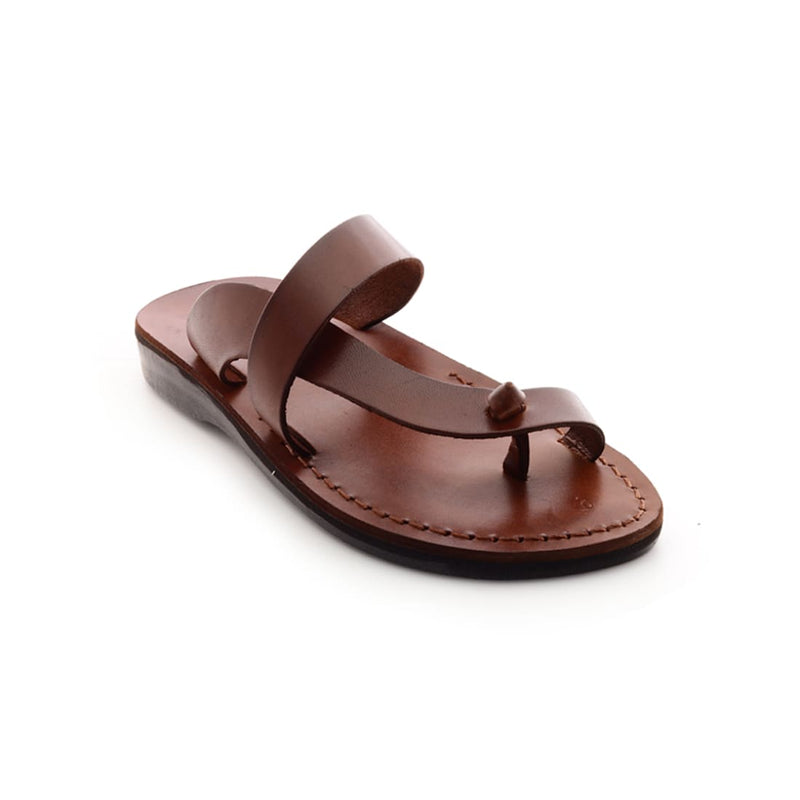This image depicts a single brown leather sandal set against a white background. The sandal features two prominent straps: one running diagonally from the top left to the bottom right, and another positioned closer to the heel, stretching horizontally from left to right. Detailed brown stitching, slightly inset from the edges, outlines the front half of the sandal. The insole shows that the straps overlap in the center, with one strap connected near the toes extending towards the heel on the outer side. A small knotted piece of leather protrudes from the front center, threaded through the front strap. The heel area of the sandal is slightly elevated, with a white section peeking out. Together, these elements create a sturdy yet simple aesthetic for the sandal.